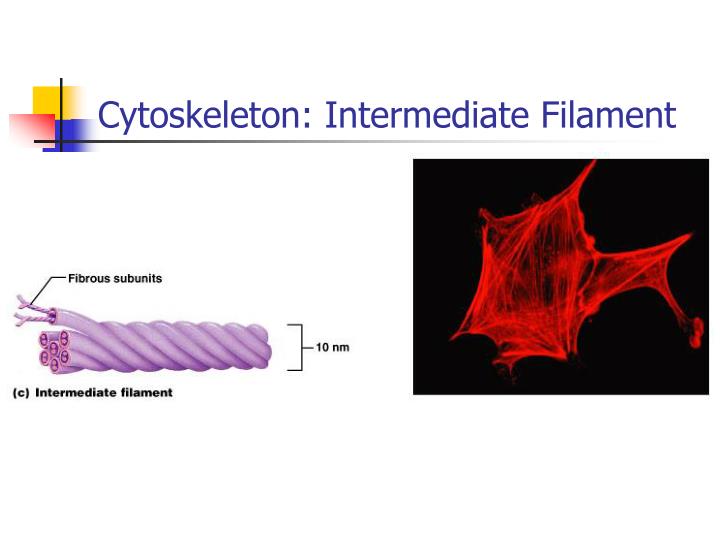This slide, seemingly from an informational scientific presentation, likely intended for medical practice, showcases the "Cytoskeleton: Colon Intermediate Filament." The slide features a title at the top, with vertical and horizontal dark-colored lines extending left to right, gradually fading. In the top left corner are three overlapping boxes in primary colors—yellow, red, and blue—that fade to white as they descend. Below the title, two images are presented. 

On the left, an illustration details the intermediate filament structure with purple coils wound together, labeled with measurements and terms such as "fibrous subunits" at the top and "C, intermediate filament" at the bottom, indicating a size of approximately 10 nanometers. 

To the right, another image, set against a black background, depicts a bright red, web-like structure, potentially representing a biological component such as a cell or neuron. The red structure appears almost transparent and stringy, suggesting intricate fibrous details. The design elements and colors used, along with the labels, emphasize the scientific and educational context of the slide, which looks as though it could be part of a textbook or a meticulous slideshow presentation.